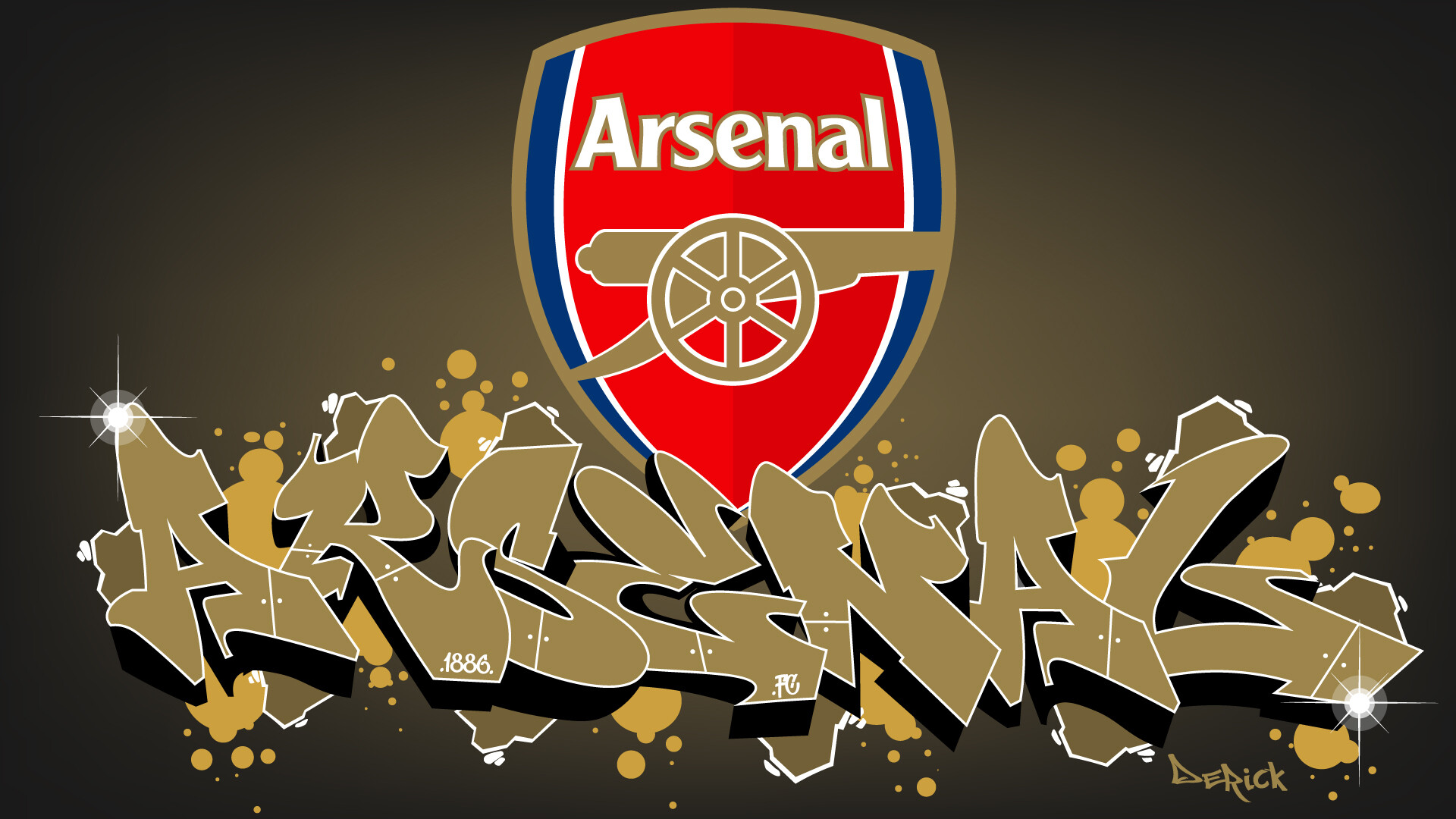The image depicts a detailed piece of wall art against a brown, metal-like background with hints of yellow paint blobs. At the center is a three-sided shield shape, featuring a predominantly red middle section outlined sequentially in white, blue, and a taupe or brownish gunmetal color. At the top of this red section, the word "Arsenal" is prominently displayed in white letters with a golden border. Beneath this, a taupe-colored cannon points to the right. Below the shield, the word "Arsenal" appears again in a graffiti-style font, creating a two-dimensional effect as if the letters are protruding from the wall. The overall aesthetic blends sports iconography with urban, street-art influences.